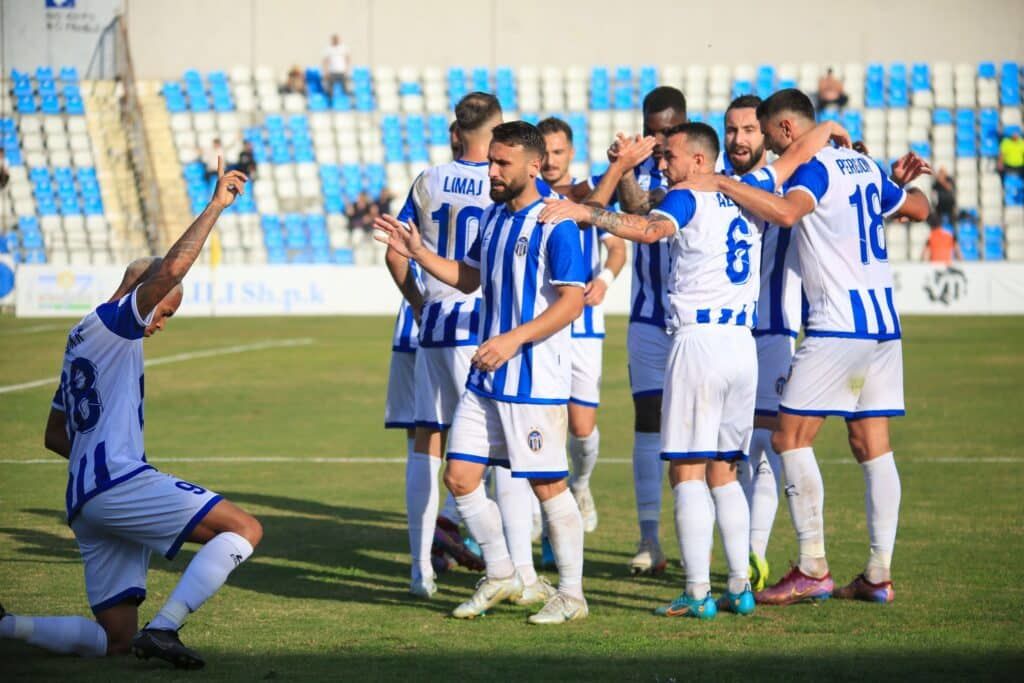In this vibrant color photograph, a group of soccer players is captured standing on a lush green field. The backdrop reveals numerous blue and white seats, sparsely populated with a few spectators. At the bottom left corner, a man is kneeling on the grass, raising his right hand with his index finger pointing upwards. He is dressed in a white and blue jersey paired with matching shorts, knee-high white socks, and soccer shoes. Dominating the center of the image is a huddling group of soccer players, all clad in blue jerseys and white shorts, complete with knee-high socks and soccer shoes. The joyful expressions and close physical proximity of the players suggest a moment of celebration. Additionally, a man is seen walking towards the kneeling player, seemingly to join in the celebration, encapsulating a triumphant and shared moment of victory.